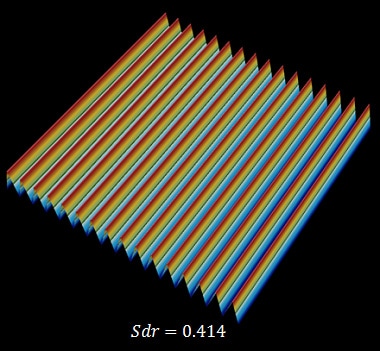The image depicts a 3D graphical representation of a series of rectangular shapes or bars standing upright and angled, set against a solid black background. Each bar features a gradient color scheme, with red at the top, transitioning to yellow, and then to light blue at the base. The bars exhibit a folded or pleated appearance, resembling the texture one might find in a window blind that can be adjusted to block sunlight. Below these shapes, white text reads "SDR = 0.414." The overall image has an abstract, almost three-dimensional quality, though it appears slightly blurry or out of focus, adding to its complexity.